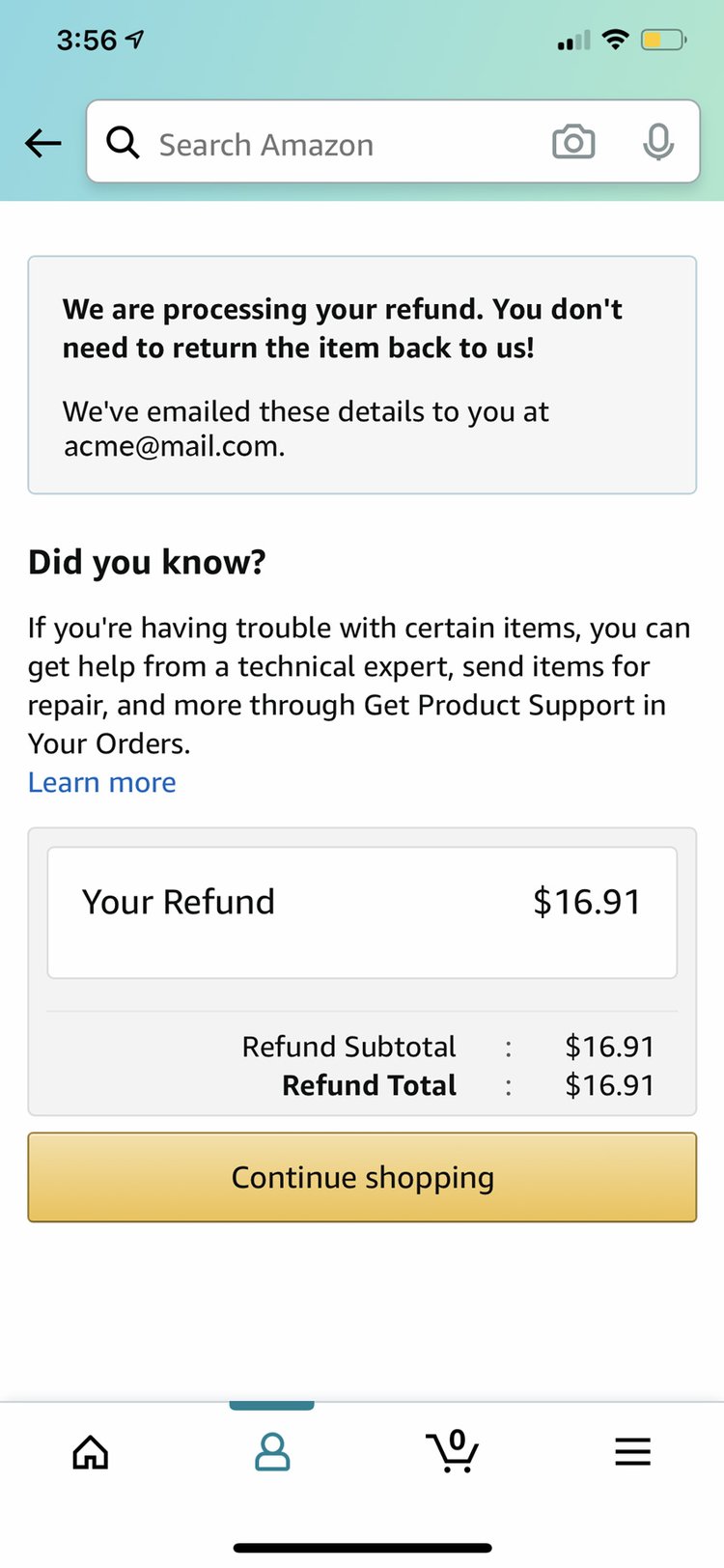In the image, we see a screenshot of an Amazon return page displayed on a smartphone. At the very top in small black text, there is a message stating, "We are processing your refund. You don't need to return the item back to us." Below this, another line informs the user, "We've emailed these details to you at acme.gmail.com."

Further down, under the heading "Did you know?", the page offers additional information: "If you're having trouble with certain items, you can get help from a technical expert. Send items for repair and more through Get Product Support in your orders."

The notification highlights that the user's refund amount is "$17 or $16.91." 

At the very bottom of the image, there is a prominent yellow button with black text labeled "Continue Shopping." This is followed by a navigation bar where the "Person" button is activated. To the left of the "Person" button is a "Home" button, while to the right, there is a shopping cart icon showing zero items and a "Settings" button at the bottom right.

At the topmost part of the page, the search bar for Amazon includes both camera and microphone icons for different search methods. Additionally, the phone’s status bar shows the time as 3:56 PM on the top left, and on the top right, icons for Wi-Fi signal strength and battery status can be seen, all set against a light blue background.